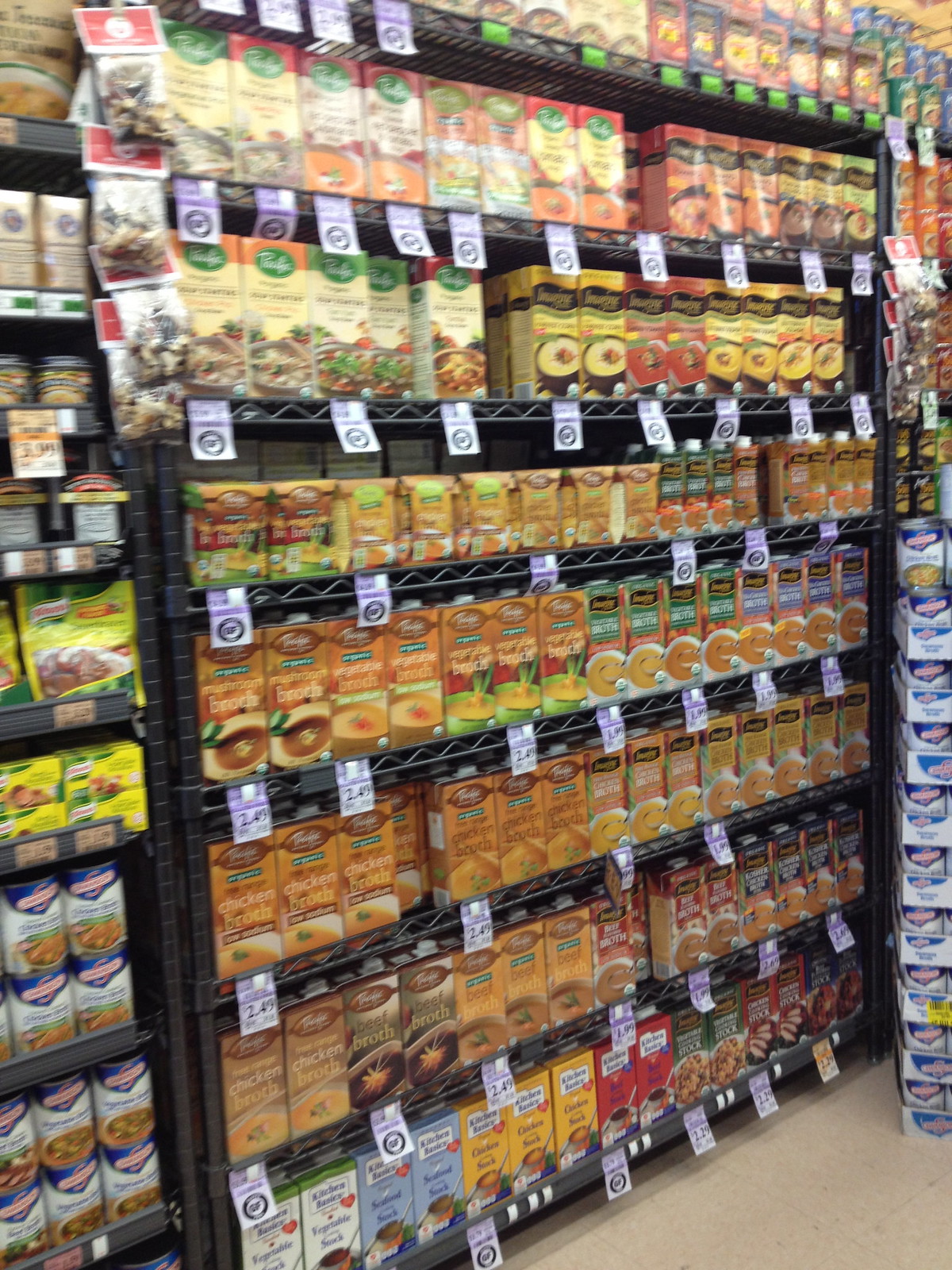A blurry photograph capturing a well-stocked store display of boxed soups, arranged predominantly in the center. The display features eight shelves, lined with colorful boxes of various soup varieties. Although the brand names are indiscernible due to the image quality, the fronts of the boxes showcase appealing pictures of soups. Small white price tags are affixed to the shelves in front of each variety. On the right edge of the photo, there's a stack of blue and white labeled canned soups, while the left side reveals another set of shelves offering additional soups and food items. The overall display implies a neatly arranged and well-maintained section, with minimal empty spaces.